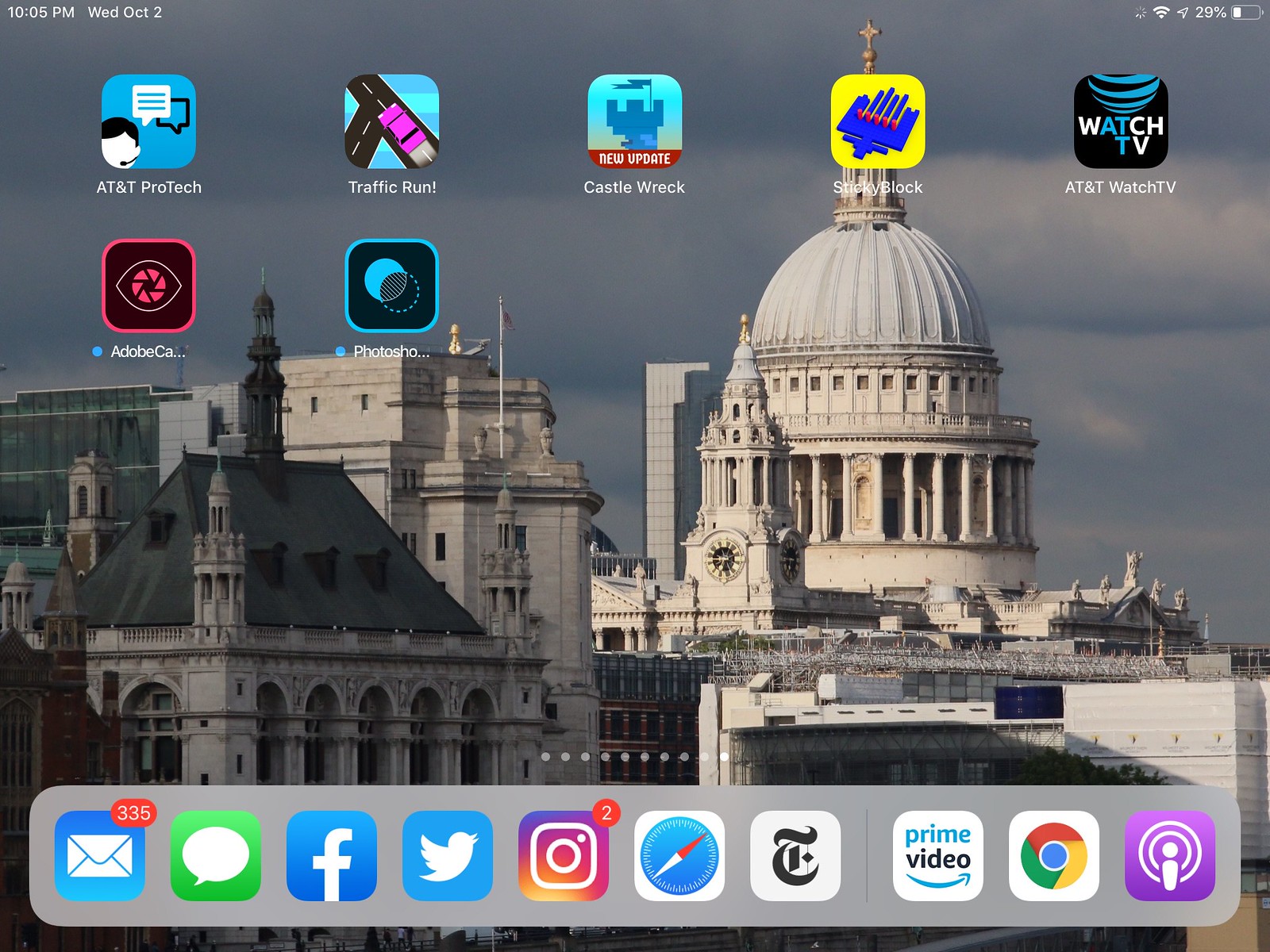The image displays various digital screens, including a computer, smartphone, and tablet, each brimming with numerous apps. A captivating screensaver adorns the background, featuring an imposing historical building resembling the U.S. Capitol, though it is not. Instead, the scene seems to represent a cityscape that might be London, given the prominent clock tower reminiscent of Big Ben and the blend of classical and modern architecture, including towering skyscrapers. The sky is a mix of dark and sunny patches, with clouds adding a dramatic tone, indicative of typical London weather.

On the desktop, various apps are visible including AT&T ProTech, Traffic Run, Castle Rec, Sticky Block, AT&T WatchTV, Adobe, and Photoshop. The taskbar at the bottom of the screen showcases icons for email, chat, Facebook, Twitter, Instagram, a compass-like symbol, The New York Times, Prime Video, Chrome, and a purple circular icon potentially representing a microphone. The assortment of applications indicates a well-rounded digital space filled with both entertainment and productivity tools.